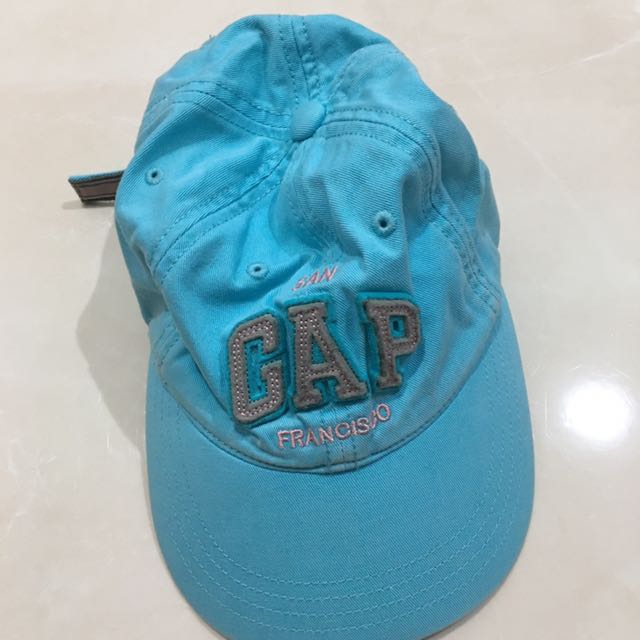The image shows a well-worn light blue baseball cap from the brand GAP, resting on a white surface. The cap features the brand name "GAP" prominently on the front in stitched, capitalized gray letters, each outlined with a thicker gray border. Just above the "GAP" logo is the word "SAN," spelled out in light pink, capitalized letters. Below the "GAP" logo, the word "FRANCISCO" is also spelled in capitalized light pink letters, completing the phrase "SAN FRANCISCO" with "GAP" in between. The cap includes three small circular ventilation holes on top. The worn appearance of the cap is noted by rough threads visible at the back, where a gray velcro strap is partially visible. Additionally, the bill of the cap appears to be white. The background of the image has a medium gray tone with subtle white lines running through it.